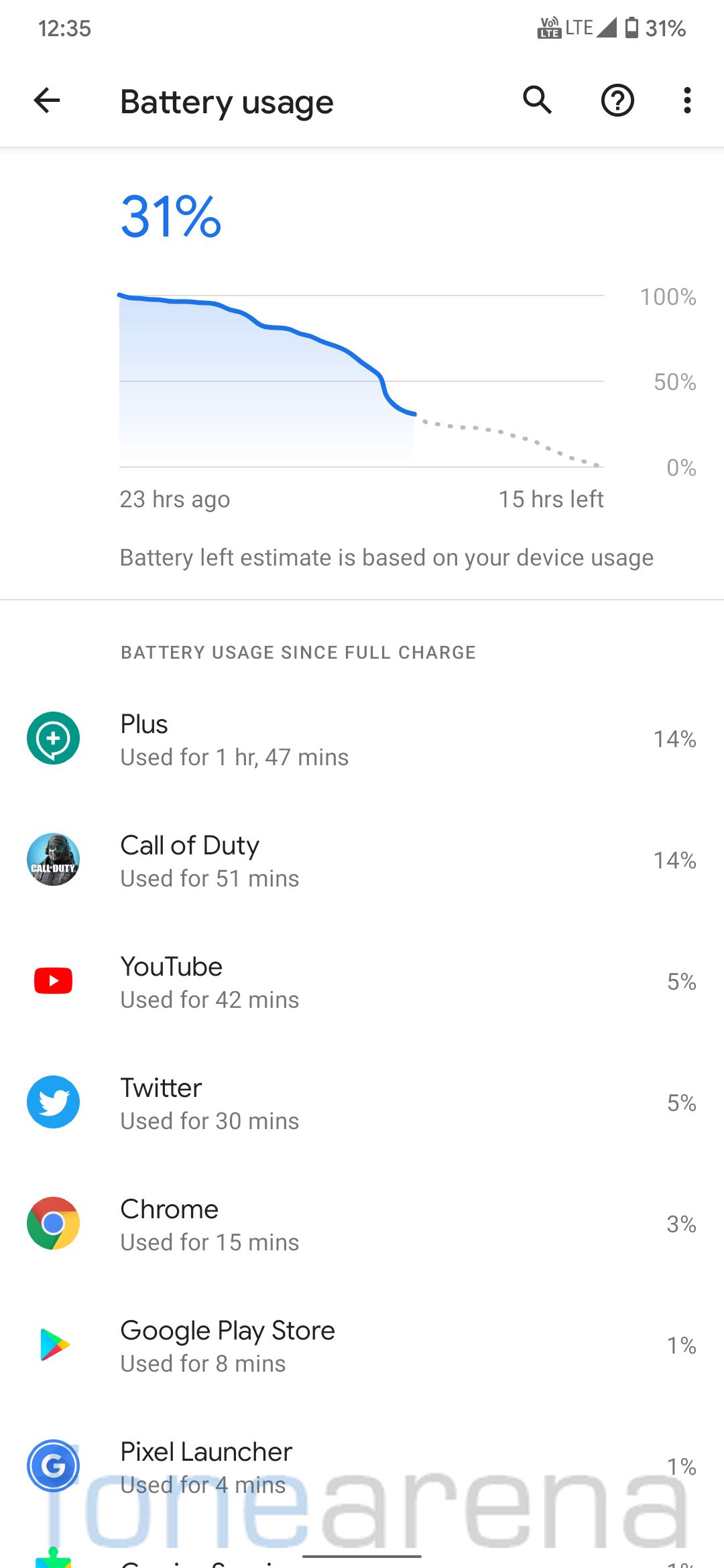The homepage screen of a user's cell phone displays detailed battery usage information. The current time at the top of the screen is 12:35, and the phone's battery level is at 31%. Below the time, the headline "Battery usage" is prominently displayed in black text. Adjacent to this text, on the right side, there are icons for search, help (question mark), and more options (three vertical dots). A back arrow icon is located to the left of the "Battery usage" text.

In the central part of the screen, a graph visualizes the battery usage over time, set against a white background with light blue elements. The top of the graph indicates the current battery level of 31% in light blue. The chart outlines battery consumption starting from 23 hours ago at a full 100% down to the current level, with markers at 50% and a noted 15 hours remaining.

Below the graph, a vertical list details battery consumption percentages since the last full charge. The list includes:
- Call of Duty: 14%
- YouTube: 5%
- Twitter: 5%
- Chrome: 3%
- Google Play: 1%
- Pixel Launcher: 1%

At the bottom of the screen, the text "One Arena" is displayed, with "One" in light blue and "Arena" in gray, forming a single concatenated phrase, "One Arena."